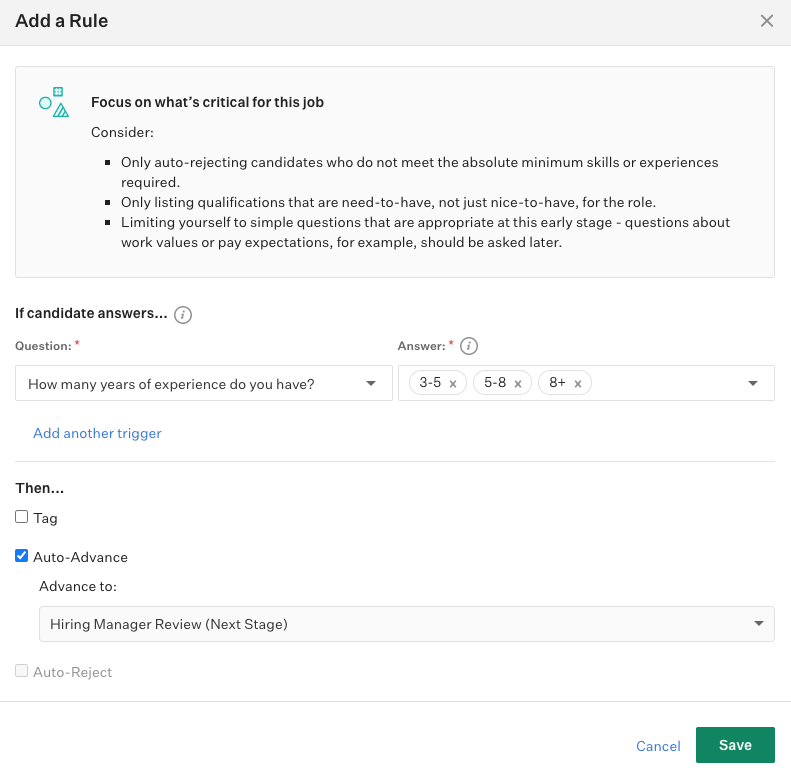The image is a detailed screen capture of an app or web page showcasing an "Add a Rule" feature. At the very top, there is a gray bar with the text "Add a Rule" and an 'X' icon in the upper right-hand corner, likely for closing the window. 

Directly below the gray bar, there is a prominent gray box featuring an icon of a blue circle, triangle, and square. This section provides important advice about setting up the rule, emphasizing that focus should be placed on essential qualifications and minimum requirements for the job. It suggests avoiding auto-rejection of candidates who meet the absolute minimum skills or experience required, only listing qualifications that are necessary rather than just desirable, and asking simple, appropriate questions at this early stage in the hiring process—reserving more detailed questions about work values or pay expectations for later.

Following this advisory section, the interface includes a decision rule: "If candidate answers question with a red asterisk next to it," with the specific query being, "How many years of experience do you have?" The possible answers listed are "3 to 5" years, "5 to 8" years, and "8+ years," each with an 'X' mark next to them to denote current selections or triggers.

Beneath this rule, there is an option to "Add another trigger" followed by the word "then..." denoting further conditional logic capabilities. Next to this is an empty box labeled "TAG," presumably for tagging or categorizing candidates based on their responses.

Further down, there's a blue box with a check mark in it labeled "Auto-advance." Below this, the text "Auto-advance to hiring manager review, next stage" clarifies the next step in the process for candidates who meet the criteria.

Finally, at the very bottom right corner of the screen, there are two buttons: a blue "Save" button and a gray "Cancel" button, allowing the user to save or discard their rule configuration.